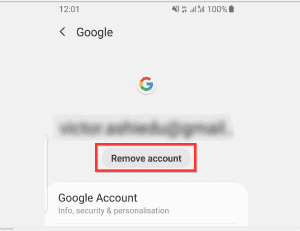The image is a screenshot taken from an Android mobile phone, as indicated by the battery percentage icon and other status indicators at the top. The battery is fully charged at 100%, and the time displayed is 12:01. The phone is on silent mode, as shown by the ringer icon. The screenshot captures a page from a Google application, likely the Google account settings or Gmail. 

At the center of the screenshot, there’s a prominent red rectangle highlighting the "Remove Account" button, signifying the user's intent to remove their Google account. Below this, text reads "Google Account," followed by sections for "Info," "Security," and "Personalization." The top left corner has a back button, suggesting navigation options within the app. Certain parts of the screen, particularly the user’s Gmail address, are blurred for privacy.